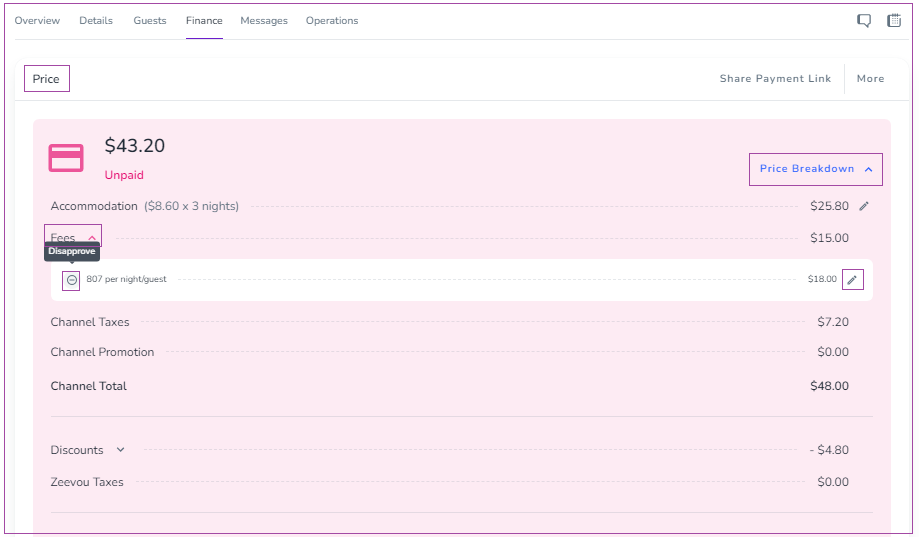The image displays an interface with several sections and details related to guest finance. At the top, there are tabs labeled "Overview," "Details," "Guests," and "Finance," with a blue underline highlighting the "Finance" tab. In the top right corner, there is an icon resembling a chat bubble labeled "Messages" and another for "Operations." Below these icons, there's a gray box with "Price" written inside, bordered by a purple outline. 

To the right, there is an option to "Share Payment Link," and just below it, several details are shown:

- Total amount unpaid is $43.20.
- Price Breakdown includes:
  - Accommodation: $8.60 per night for three nights.
  - Fees: $8.07 per night per guest.
  - Guest Fees: $18.
  - Channel Fees: $15.
  - Taxes: $7.20.
  - Channel Promotion: $0.
  - Total Channel: $48.
  - Discounts: -$4.80.
  - Guests: "Ziva", "Zivo", "Z ee vo" are listed.
  - Taxes: $0.00.
  
The background of the image is pink except for the section detailing "8.07 per night/guest," which has a white background and is bordered by a thin pink line around the entire image.